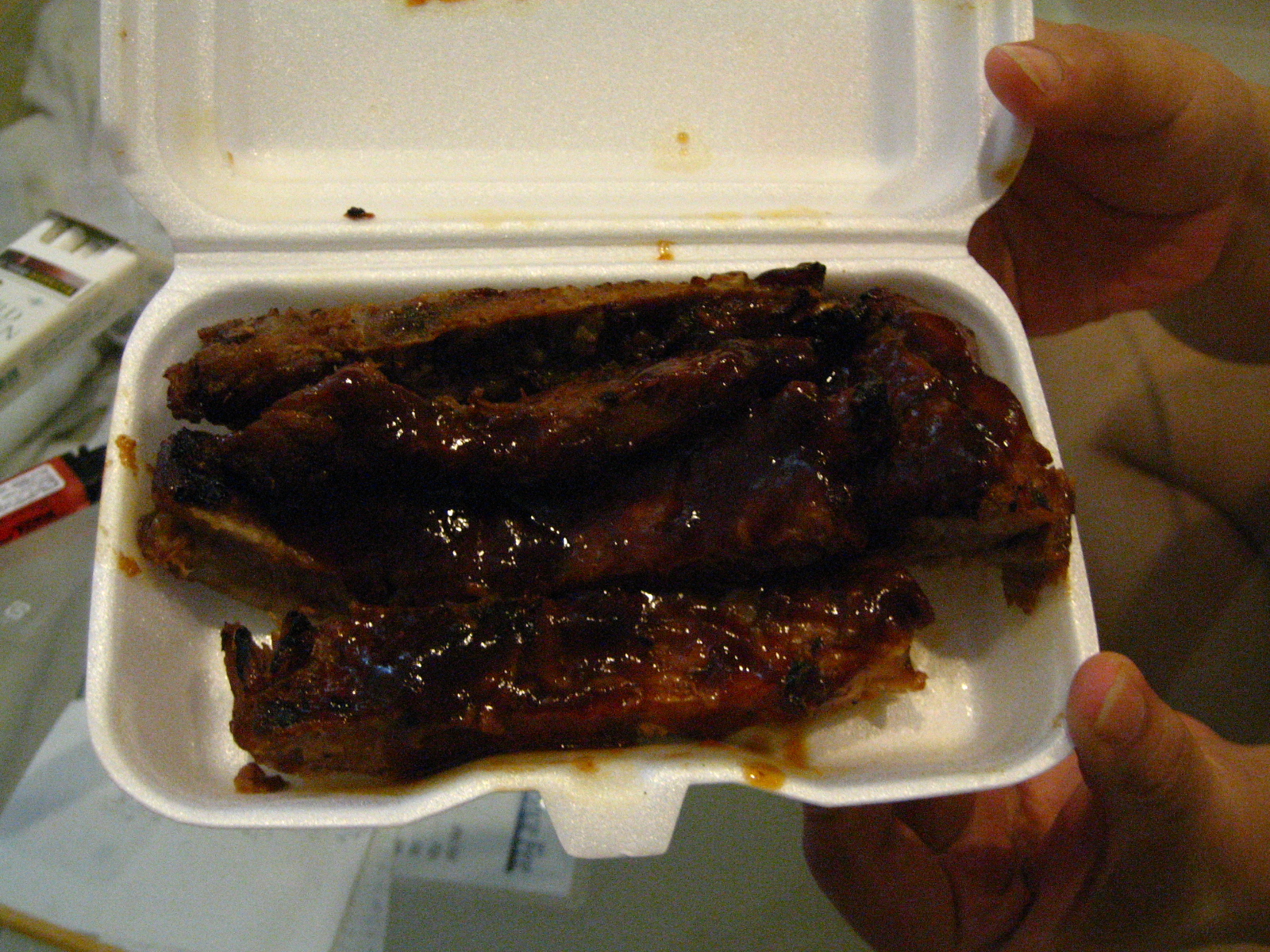This photograph captures a man of European descent holding open a rectangular styrofoam takeout tray with a built-in tab. Inside the tray, there are approximately six long, narrow pieces of bone-in ribs, each roughly six inches in length. The ribs are well-cooked, brown, and glazed with a thick, deep red barbecue sauce, with some torn bits apparent. The man is displaying the tray to the camera. In the background, on what appears to be a table, there is a pack of cigarettes and a lighter, alongside several papers, possibly including a laminated card or pass. The setting appears to be indoors, perhaps near a refrigerator based on the lighting.